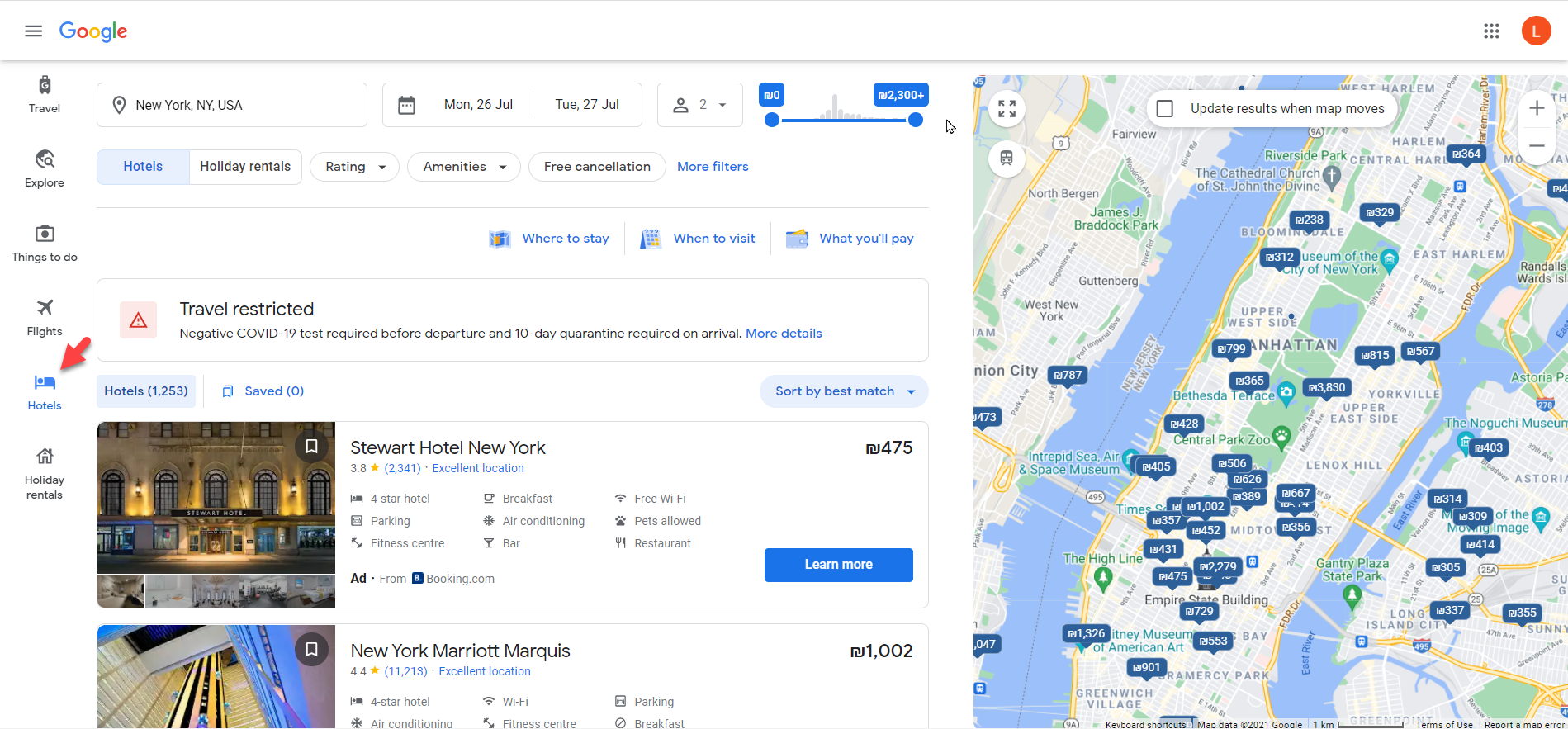The image depicts a Google search results page for a travel query to "New York, New York, USA". At the top of the page, a text box contains the search location alongside a calendar icon, indicating travel dates from Monday, 26th July to Tuesday, 27th July. Adjacent to this, a dropdown menu displays a person icon with the number 2, likely representing the number of travelers.

Below this search section, there are tabs labeled "Holiday", "Hotels", "Holiday Rentals", "Ratings", "Amenities", and "Free Cancellation". The "Hotels" tab is currently highlighted.

Further down, informational headers are visible with the titles "Where to stay", "When to visit", and "What you'll need". Following this, a warning box appears stating travel restrictions: "Negative COVID-19 Tests Required Before Departure" and a "10-Day Quarantine Required On Arrival".

In the hotel listings below, the "Stewart Hotel, New York" is featured with a 3.8-star rating from 2,341 reviews. Descriptions indicate it as an "Excellent Location, 4 Star Hotel" offering amenities such as "Parking, Fitness Center, Breakfast, Air Conditioning, Bar, Free Wi-Fi, Pets Allowed, and Restaurant". A blue button labeled "Learn More" invites users to obtain additional details.